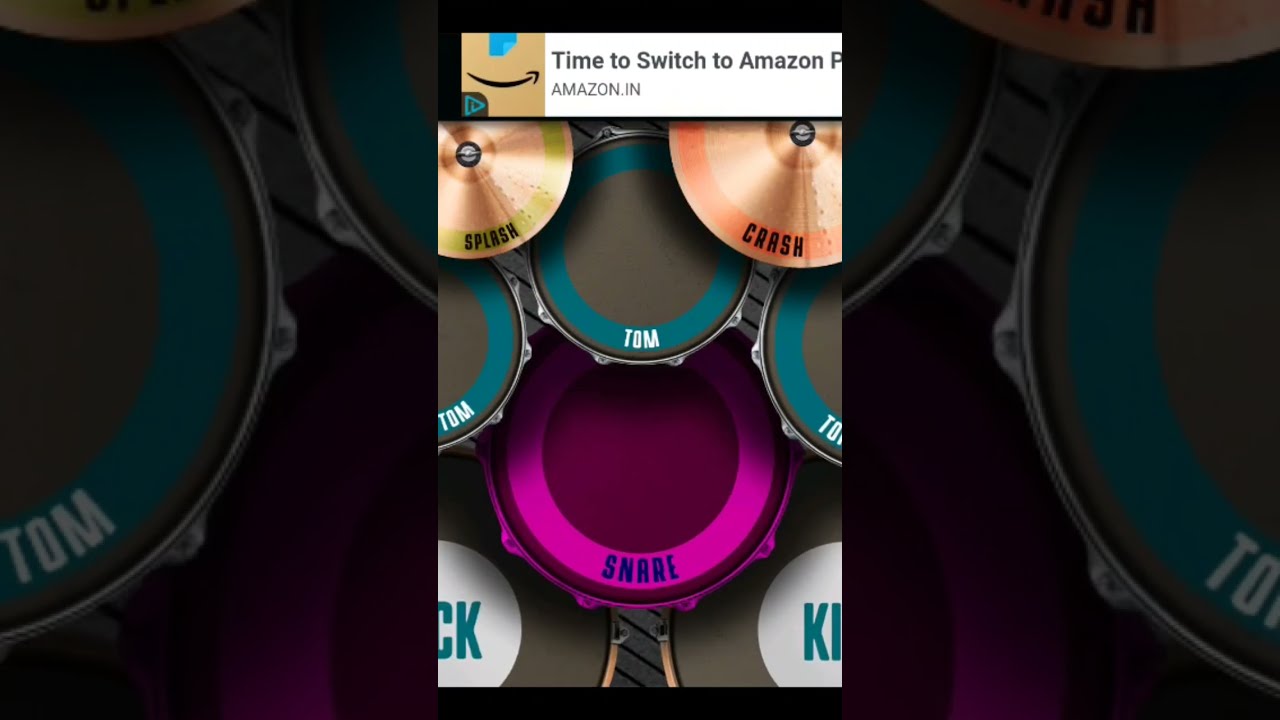The image, possibly a screenshot taken on a smartphone app, features a simulated drum set within a vertically cropped frame. At the top of the image, an ad banner reads "TIME TO SWITCH TO AMAZON" with a URL "AMAZON.IN," set against a white rectangular background and accompanied by the familiar brown Amazon logo with its smiley face swoop. 

Below the banner, the drum set is displayed, with various drum pads and cymbals labeled clearly. The snare drum, centrally positioned, is enclosed in a pink circle and marked with purple writing that reads "SNARES." Surrounding the snare are three tom drums, each encased in a light blue-teal circle, and labeled "TOM" in white writing. 

To the top left and right are the cymbals: a "SPLASH" cymbal on the left in a green circle with black lettering, and a "CRASH" cymbal on the right in an orange circle with black lettering. At the bottom of the image, two larger drum pads labelled "KICK" are present, though partially cropped, showing "CK" on the left and "KI" on the right, each within a white circle.

The image's center section is lighter, with the left and right edges displaying a darker, zoomed-in version of the drum set, featuring shadow effects adding depth. The overall layout and labeling, enhanced by various colors and clear demarcations, suggest a detailed and interactive design typical of a drumming simulation game or app.